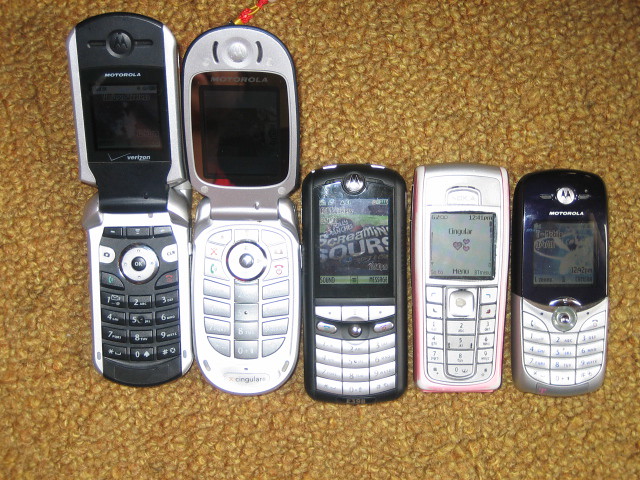This photograph depicts five vintage cell phones neatly laid out on a textured Berber carpet, which is a blend of beige, orange, and yellow hues. The first two phones on the left are classic Motorola flip phones, opened up to reveal their screens and keypads. The first flip phone prominently displays the Verizon logo at the bottom of its screen. Moving right, the third phone is a candy bar style phone with a barely visible 'M' logo at the top, likely indicating it's also a Motorola. The fourth phone, darker in color, appears similarly styled as a candy bar phone, while the fifth distinctly shows the Motorola branding, featuring a black upper section and a gray keypad area. Scattered amongst the details of the phones, there's a noticeable small red bead either resting on the carpet or possibly attached to the second flip phone. The overall scene is set against the warm, inviting tones of the carpet, emphasizing the nostalgic feel of these early 2000s mobile devices.